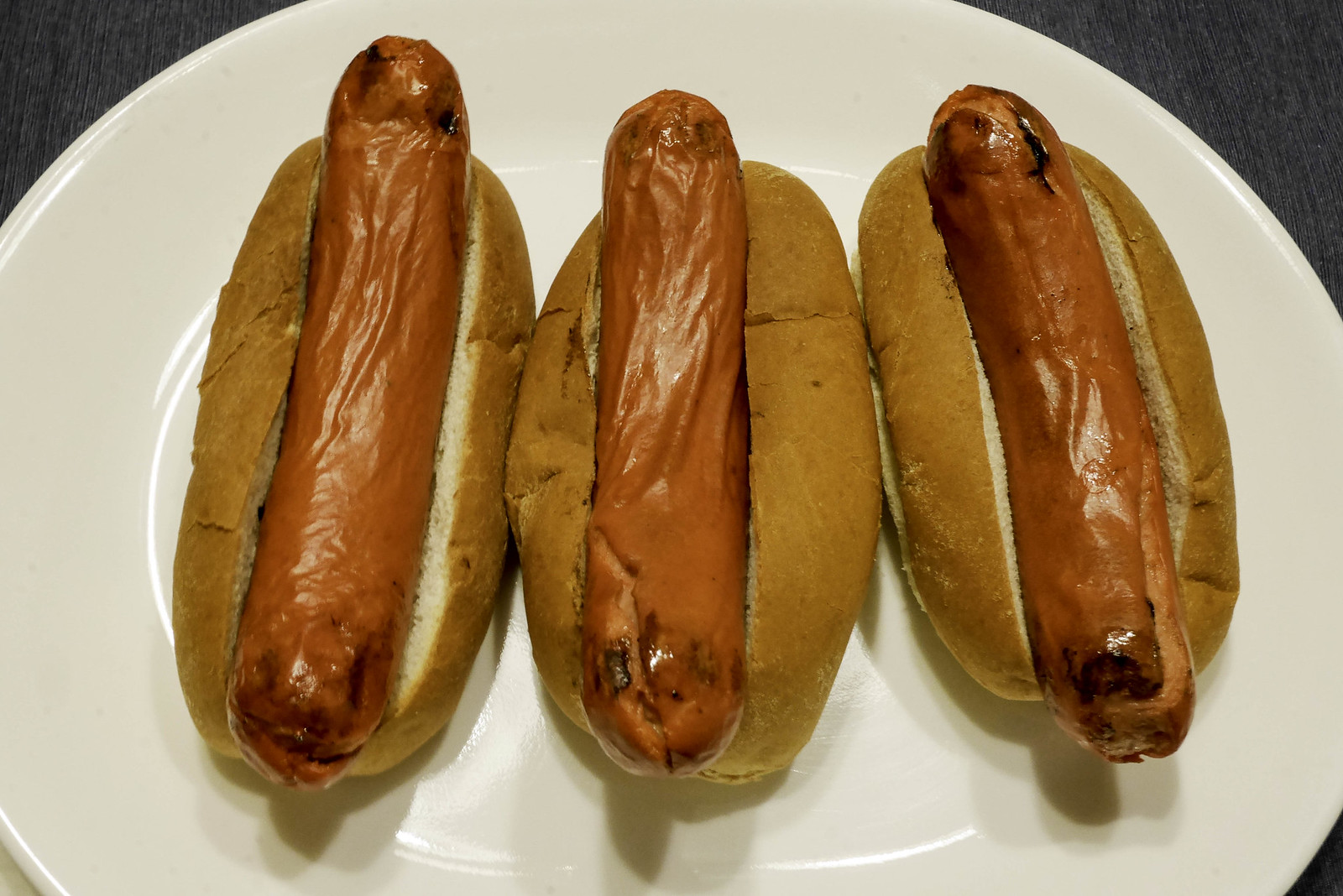A close-up, colored flash photograph captures three hot dogs in buns on an oval-shaped, white ceramic plate. The plate sits on a gray wooden table, evident from the fine grain visible in the background, although the edges of the plate are cropped from the image, leaving a black backdrop beyond. Each hot dog is lined up horizontally from left to right, with the hot dogs themselves vertically aligned. The buns have a dark brown exterior and a white interior, appearing flat and somewhat stale. The hot dogs, medium brown in color with black char at both tips, look shriveled and wrinkly, as if overcooked or aged. Highlights on their wrinkled skin suggest reflections from the overhead lighting. Despite the pale pink-brown hue indicative of typical hot dogs, their excessively wrinkled, crinkly appearance makes them look unappetizing, almost as if their skin could peel off. The plate and hot dogs reflect the light source above, casting slight shadows at the bottom, with no condiments or additional garnishes visible.